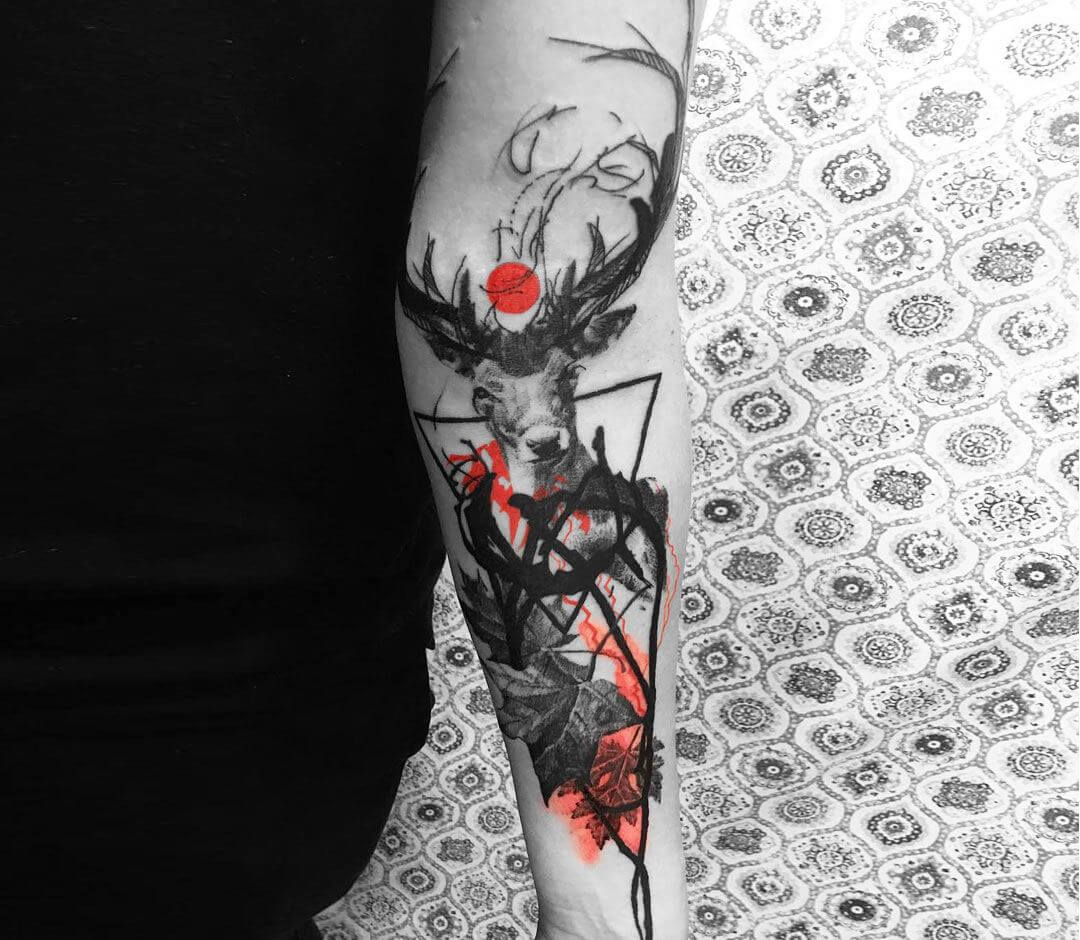In this photograph, the viewer's attention is drawn to the intricate tattoo on the back of a person's arm. The individual is mostly off-screen, with only their arm and a portion of their torso visible, clad in a sleek black outfit. The floor beneath them features a striking black and white geometric pattern, adding a dynamic backdrop to the scene. The central focus, however, is the exquisitely detailed tattoo of a deer head on the person's arm. The deer, facing forward, boasts long, elegant antlers that curve upward and outward in a graceful arc. Surrounding the deer's head is a complex geometric design interwoven with thick black lines and delicate leaf motifs. Adding a striking contrast to the predominantly black and white tattoo, a vivid red circle is positioned above the deer's head. Additionally, hints of red blur near the bottom of the image, enhancing the visual impact of the photograph.